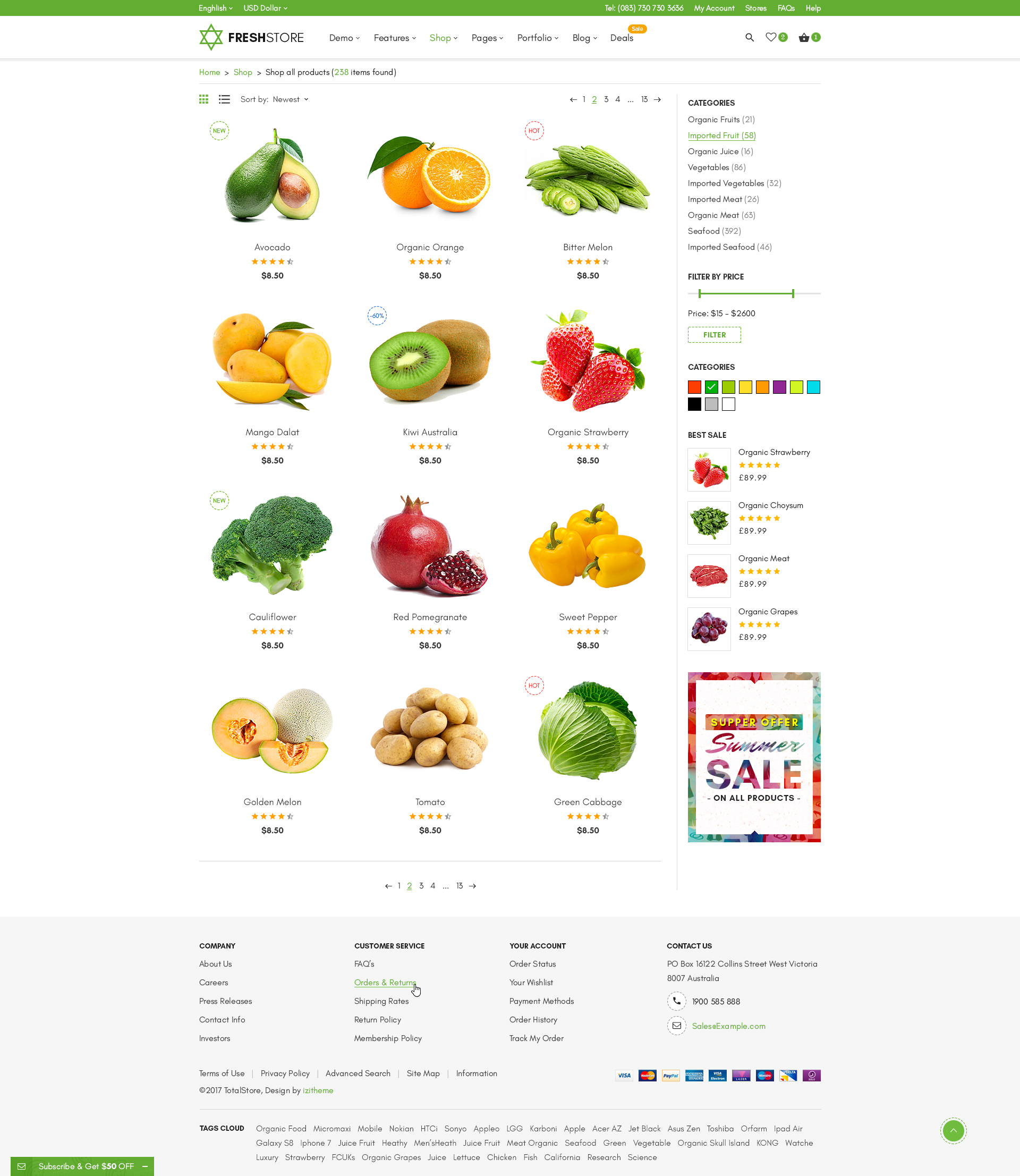This vibrant image depicts the homepage of an online fruit and vegetable store named "Fresh Store." The website's design features a full-page layout adorned with brightly-colored images of various fruits and vegetables, enhancing its visual appeal. The store's logo, prominently displayed, resembles a star formed by an upwards-facing and downwards-facing triangle stacked together.

The product display begins with a perfectly ripe avocado, its price clearly visible underneath. Adjacent are plump oranges, with one fully intact and another halved to reveal the juicy segments inside. The assortment of produce continues with cucumbers, lemons characterized by their thick yellow rinds and green leaves, and kiwis—brown and fuzzy on the outside, green with a white center on the inside. Also featured are vibrant red strawberries with lush green leaves, and a lush green broccoli that resembles a miniature tree.

A pomegranate, vivid red on the outside and filled with jewel-like edible seeds inside, adds to the variety. Bright yellow peppers in their characteristic shape, pumpkins, earthy potatoes, and a leafy green cabbage round out the selection, providing a comprehensive view of the store’s diverse offerings.